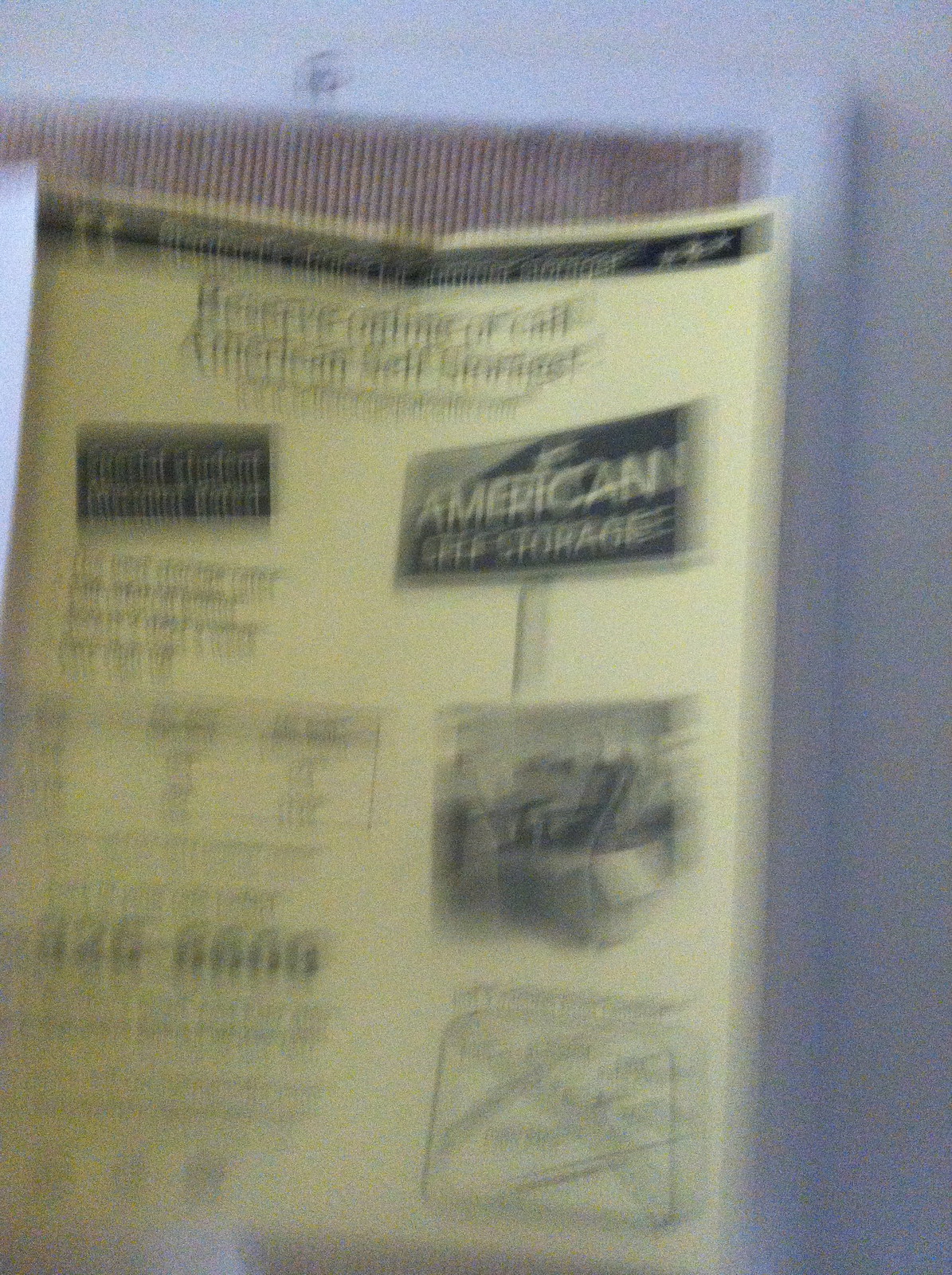This image captures a sign that appears to have been photographed under low light conditions, resulting in significant blurriness. The sign itself is printed on yellow paper with black text and includes several distinct sections. At the top of the sign, the text reads "Reserve Online or Call, American Self Storage." Directly below this, there is additional text that is too blurry to decipher. Beneath this section, there is a black square with yellow text, which is also unreadable due to the blur. The middle part of the sign displays a billboard image that reads "American Self Storage," accompanied by what seems to be a black-and-white photograph of chairs. Towards the bottom of the image, there appears to be a section resembling a map with directions, but it, too, is extremely blurry and indistinct. A phone number is partially legible: it could be either "3" or "8," followed by "2," "5" or "6," and ending in "8808." Despite the overall lack of clarity, the sign's purpose appears to be promoting American Self Storage services.